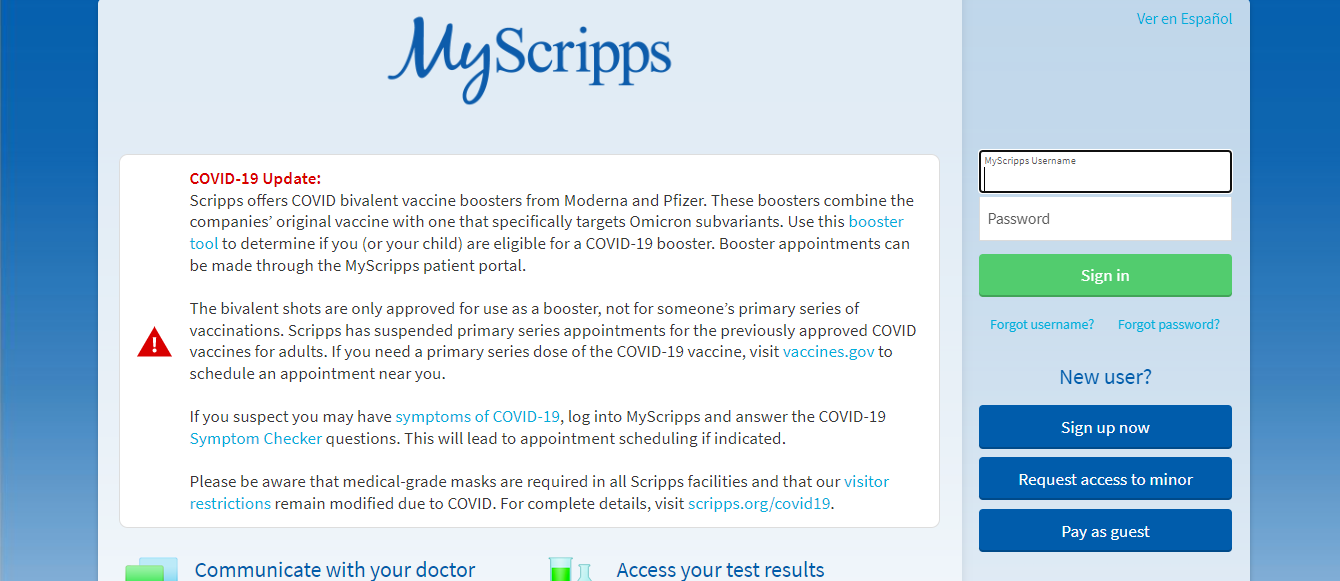This image is a screenshot of the MyScripps patient portal login page, prominently featuring a COVID-19 update. 

At the top, the page displays the MyScripps logo in blue text. In the top-right corner, there is a link labeled "Ver en Español" for the Spanish version of the page. A critical COVID-19 update is highlighted in bold red text. The update informs users that Scripps is offering COVID-19 vaccine boosters from Moderna and Pfizer, specifically targeting Omicron sub-variants. Users can check their eligibility for a booster using a linked booster tool. Key points include that Bivalent shots are only for boosters, not for the primary vaccination series, which Scripps has suspended for adults. For primary series doses, users are directed to visit vaccines.gov. Those suspecting COVID-19 symptoms are advised to log into MyScripps and use the COVID-19 symptom checker. The update also notes that medical-grade masks are mandatory in all Scripps facilities and that visitor restrictions are enforced.

Below the update, there are several links including: 
- Booster Tool
- Vaccines.gov
- Symptoms of COVID-19
- Symptom Checker
- Visitor Restrictions
- Scripps.gov/COVID-19

On the right side of the page, the login section prompts users for their MyScripps username and password. There are green buttons for "Sign In" and hyperlinks for "Forgot Password" and "Forgot Username." Below this, a prompt for new users features three large blue buttons labeled "Sign Up Now," "Request Access to Minor," and "Pay as Guest." At the bottom, there is an additional note stating "Communicate with your doctor and access your test results."

This detailed overview captures the essence and functionality of the MyScripps patient portal login page as seen in the screenshot.